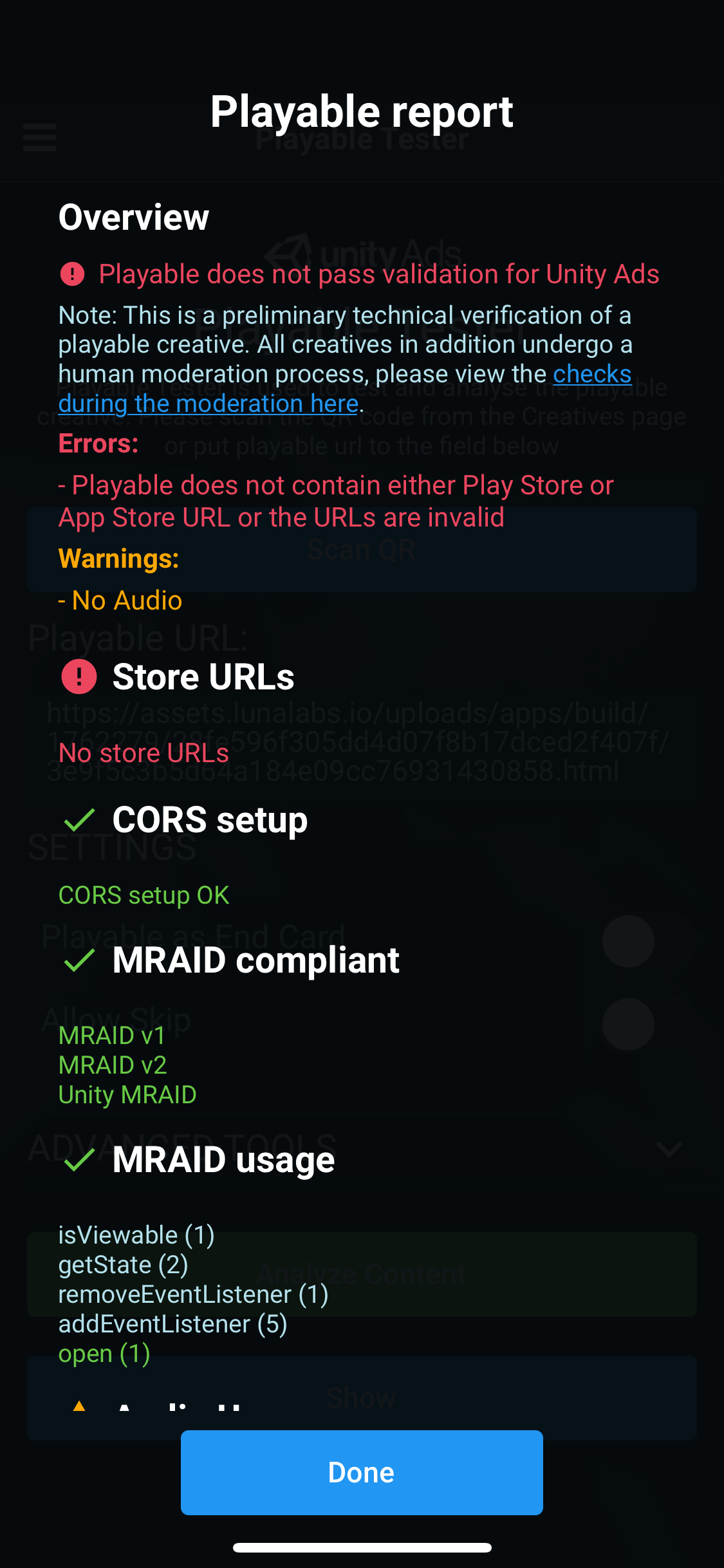The image depicts a desktop screenshot featuring a predominantly black background. At the top-middle of the screen, "Playable Report" is prominently displayed in white letters. Below this heading, on the left side, "Overview" is highlighted in red letters, followed by an alert in white text stating, "Playable does not pass validation for Unity Ads."

A light blue note below this alert provides additional information: "This is a preliminary technical verification of a playable creative. All creatives also undergo a human moderation process. Please view the checks during the moderation here." The phrase "checks during the moderation here" is hyperlinked, underlined, and colored blue, suggesting it leads to another page when clicked.

Further down, a red error message indicates: "Playable does not contain either Play Store or App Store URL, or the URLs are invalid." An orange warning beneath it states: "No audio."

Additional sections include:
- **Store URLs:** Highlighted in red with an alert stating "No store URLs."
- **CORS Setup:** Accompanied by a green checkmark and the message "The CORS setup is okay."
- **M-RAID Compliant:** Marked with a green checkmark, followed by green text listing "M-RAID V1, M-RAID V2, Unity M-RAID."

At the very bottom of the page, a rectangular light blue button labeled "Done" is centered.